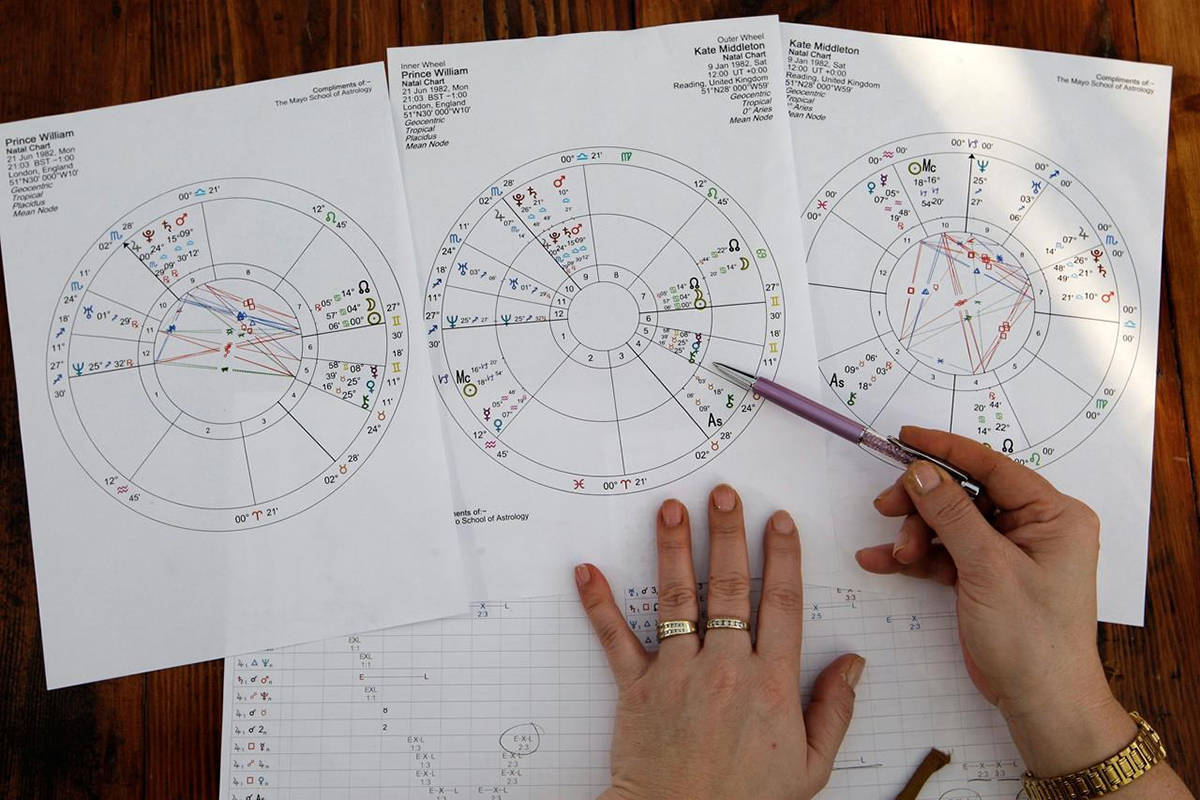The photograph captures a detailed scene of someone analyzing astrological natal charts on a desk. The focus is on the person's hands, which are adorned with gold rings on the left hand and a gold watch on the right wrist. The right hand holds a purple pen. Spread across the desk are three overlapping sheets of paper, each displaying a detailed astrological wheel diagram. The charts are labeled "Prince William," "Prince William and Kate Middleton," and "Kate Middleton," and contain intricate symbols, numbers, and colorful sections, likely related to astrological readings. The papers appear to come from the Mayo School of Astrology and are dated January 9, 1982. The person's pen is pointing thoughtfully at one of the charts, suggesting they might be examining the compatibility between Prince William and Kate Middleton. Additional partially visible papers and sunlight add depth to the scene, emphasizing the studious and analytical atmosphere.